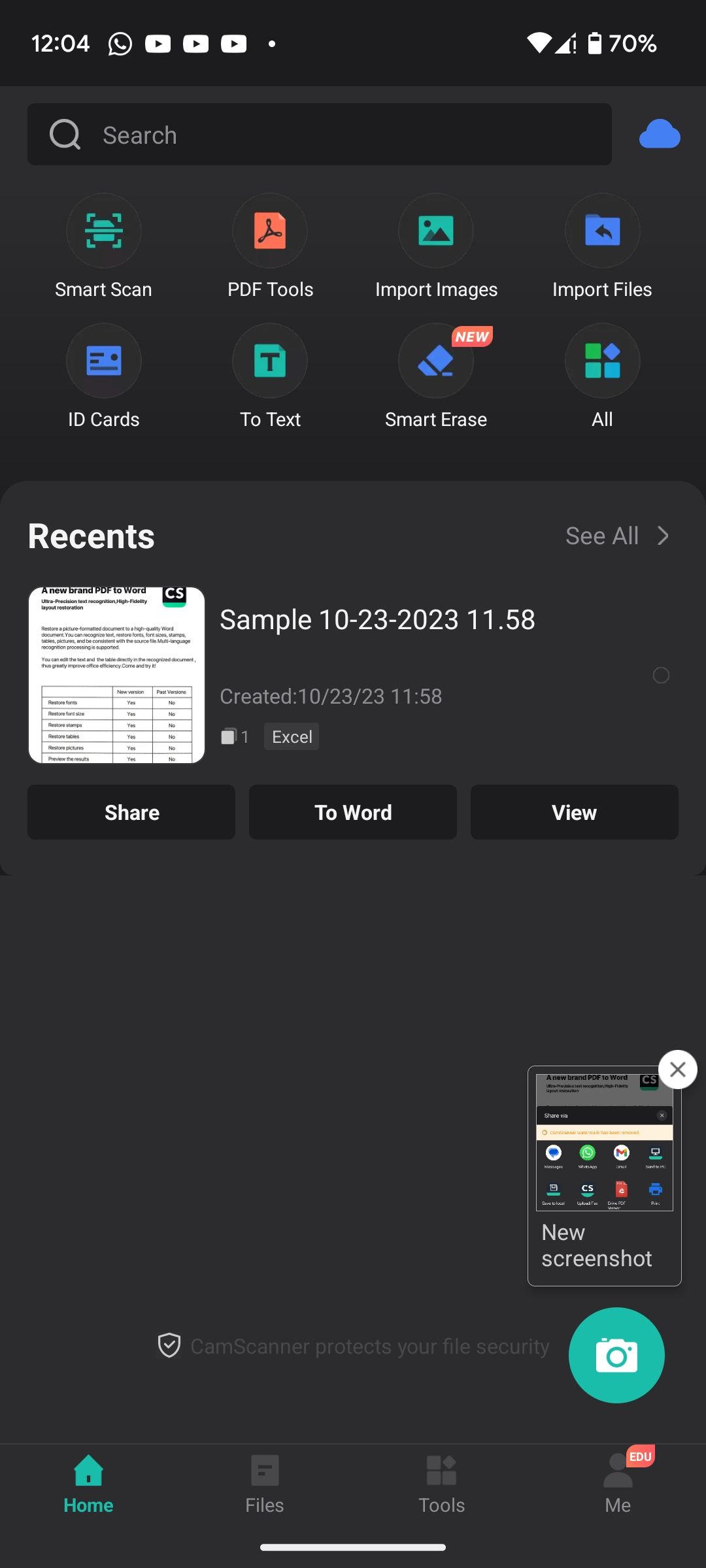**Screenshot Description:**

The screenshot captures a mobile device's display with various app icons and interface elements. 

**Top Section:**
- **Status Bar (Top Left Corner):** The time displayed is 12:04. Nearby, there are icons for WhatsApp and three YouTube accounts.
- **Status Bar (Top Right Corner):** The Wi-Fi icon is active, and the battery is at 70%.

**Middle Section:**
- **Search Bar:** Below the status bar, a search bar with the text "Search" is visible. To the right of the search bar is a blue cloud icon.
- **App Interface Options:**
  - Several action buttons are arranged horizontally, which include:
    - "Smart Scan"
    - "PDF Tools"
    - "Import Images"
    - "Import Files"
    - "ID Cards"
    - "To Text"
    - "Smart Erase"
  - Beneath these buttons, options such as "All," "Recents," and "See All" are listed.

**Document Information:**
- A file named "sample" with metadata is showcased:
  - **Filename:** "sample 10-23-2023 11.58"
  - **Creation Time:** "created 10-23-23 11.58"
  - **File Type:** Excel document.
  - To the left, a preview snippet of the document is shown with the header "A New Brand PDF to Word," followed by options to "Share to Word" and "View."

**Notification:**
- A notification bubble with the text "New screenshot" is also present on the screen.

**Bottom Section:**
- A footer message reads: "CamScanner protects your file security."
- A navigation bar at the bottom includes icons for:
  - **Camera**
  - **Home**
  - **Files**
  - **Tools**
  - **Me**

**Overall Image Proportions:**
- The image has a portrait orientation, being taller than it is wide.

This description captures the detailed elements and layout of the screenshot taken from a mobile device, providing a clear understanding of the visual content and app interface.